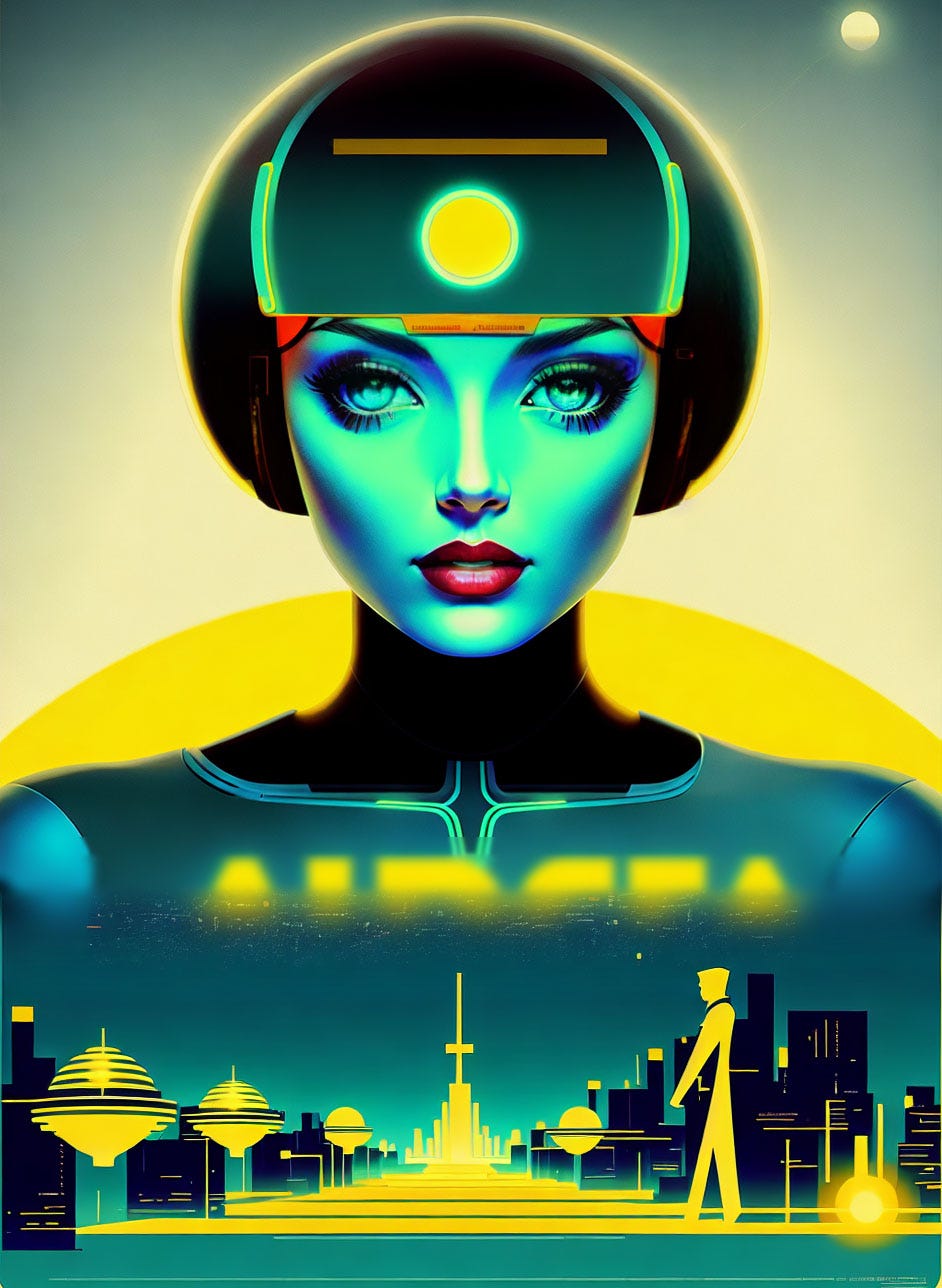The image features a highly detailed, AI-generated depiction of a futuristic woman with striking, exaggerated features that give off a movie poster vibe. Her skin is illuminated in shades of green and blue, with a neon green light highlighting her face and darker blue tones adding depth. She has large, heavily mascaraed blue eyes, a small, perfect nose, and bold red lips. Her black bob haircut completes her modern appearance, and she wears a high-tech helmet with a bright yellow light at the center of her forehead.

Her attire resembles a sleek, metallic spacesuit with black shoulders and sections, adorned with yellow lettering that is partially visible. The lower portion of the image showcases a futuristic cityscape in a palette of yellow, black, and blue. This scene includes silhouettes of tall buildings, illuminated orbs, and flying saucer-like objects, all centered around a man walking along a path under a yellow glow. The overall aesthetic is very robotic and cyberpunk, encapsulating a vision of a high-tech, alien-like future.